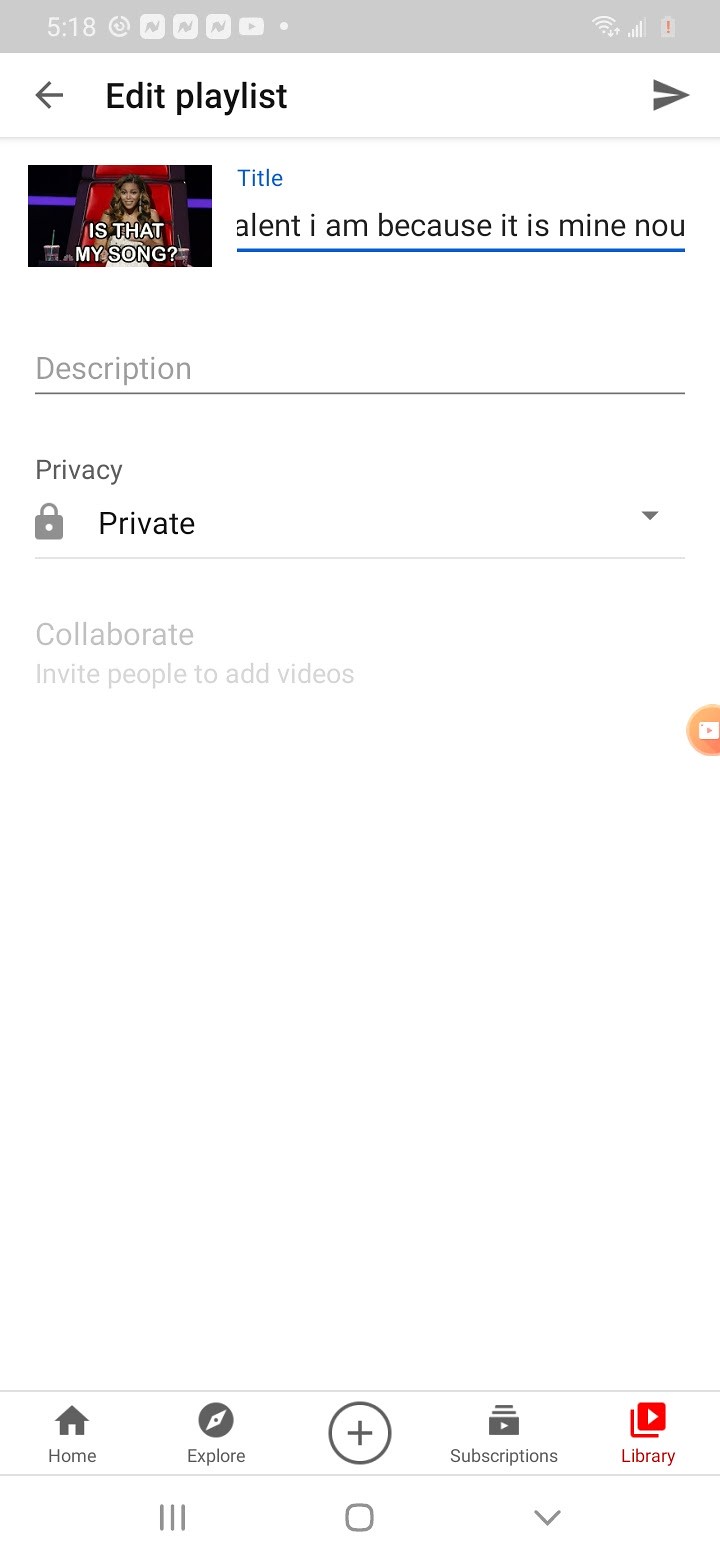This image depicts a screenshot of a mobile device displaying a YouTube playlist editing interface. At the top of the screen, the status bar displays several icons: the time (5:18), a power/battery saver icon, a News Break app icon, a YouTube app icon, and a white dot. On the right side of the status bar, the Wi-Fi signal strength, cellular signal strength, and a battery icon with a red exclamation mark indicating low battery are visible.

The main section of the screen shows the "Edit Playlist" interface. At the top of this section, there is a left-facing arrow, followed by the text "Edit Playlist" in black. To the right, there is a triangular send arrow typically used in messaging apps. Below, there is an image that seems to feature a contestant from the show "The Voice." The contestant appears to be an African American woman with long, curly hair and baby hairs styled along her hairline. She is seated in one of the show's iconic chairs and holds a clear cup with a straw in her right hand. 

Next to the image, the text "Is that my song?" is present along with the partial title "ALENT," suggesting the title might have been cut off ("TALENT" inferred). Below the title, a blue line indicates a text input field followed by the word "Description" in gray. Underneath, there is a "Privacy" section with a lock icon and the label "Private" accompanied by a drop-down arrow. Further down, a grayed-out option labeled "Collaborate: Invite people to add videos" indicates that collaboration is not currently enabled.

On the right side of the interface, there is a semi-circle icon with a white square and an orange play arrow inside it, implying a media play function. The lower part of the screen shows the YouTube navigation bar with icons for Home, Explore, Add (a circle with a plus sign), Subscriptions, and Library (the Library icon is highlighted in red). Below these icons are navigation controls: three lines, a square, and a down arrow, which are typical for Android devices to access recent apps, go back, or return to the home screen.

This detailed description clarifies that the screenshot is from a YouTube app, specifically within a playlist editing feature.